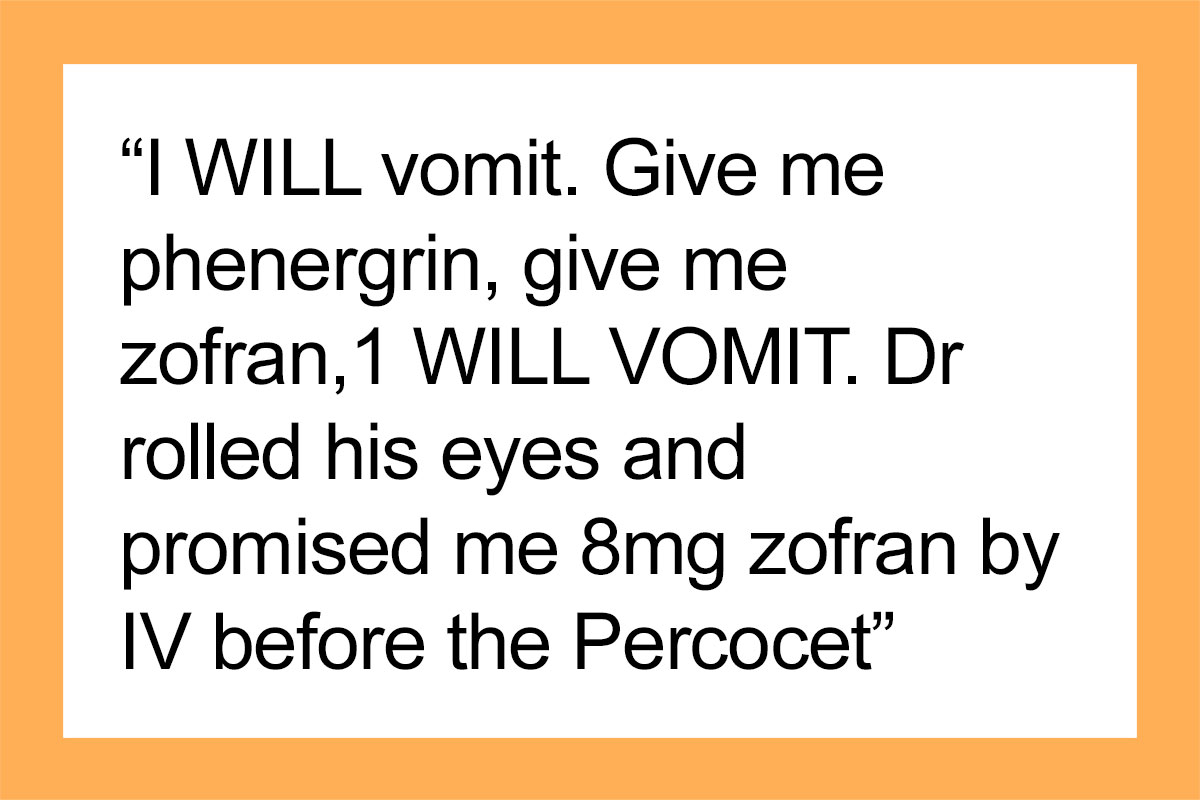The image depicts a sign with a narrow, light-orange (or yellowish peach) border surrounding a large white background. Centrally featured in bold black Arial text, the sign proclaims in various capitalizations: "I WILL VOMIT. GIVE ME PHENERGAN, GIVE ME ZOFRAN, I WILL VOMIT, WILL VOMIT." It continues with: "Doctor rolled his eyes and promised me 8 milligrams Zofran by IV before the Percocet." The text is arranged without any periods. There are no other graphical elements besides the described text and border, possibly suggesting the content could come from a PowerPoint presentation or a similar format.